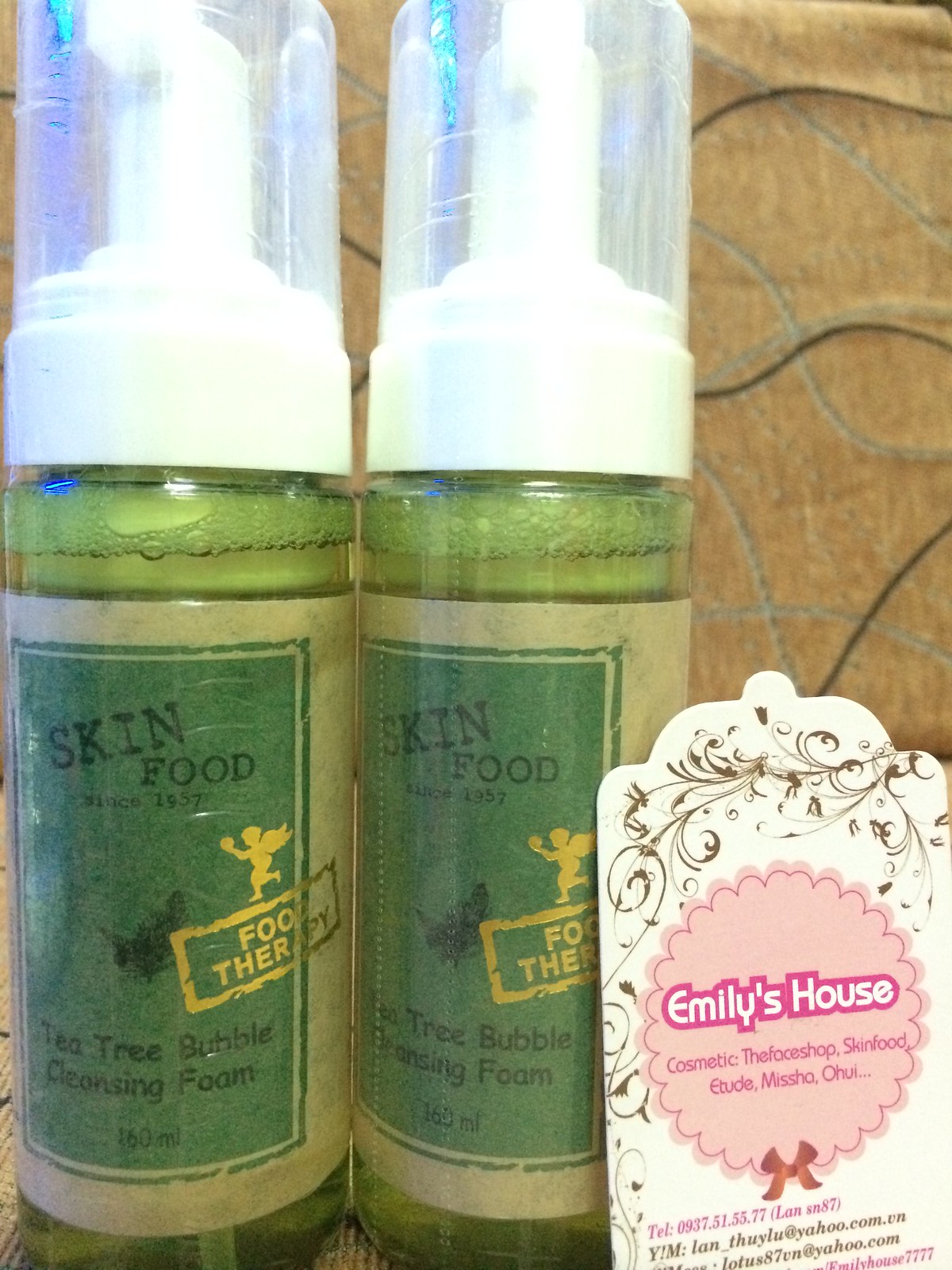This is a close-up photograph of two green bottles of skin care product, specifically Tea Tree Bubble Cleansing Foam by Skin Food. Both bottles feature white pump applicators on top. The labels, predominantly green, include the brand name "Skin Food" in black text and a small gold cherub with the words "food therapy" beneath it. Each bottle contains a green bubbly liquid, indicated on the labels as 160 milliliters. Positioned to the right of the bottles is a decorative card adorned with brown filigree and a yellow or pink floral shape in the middle. This card reads "Emily's House Cosmetic" and lists additional cosmetic brands such as The Face Shop, Etude, Missha, and Ohui. The photograph appears to be taken in a store or shop with a beige background that has lines running through it, emphasizing the central focus on the two prominently displayed cosmetic bottles.